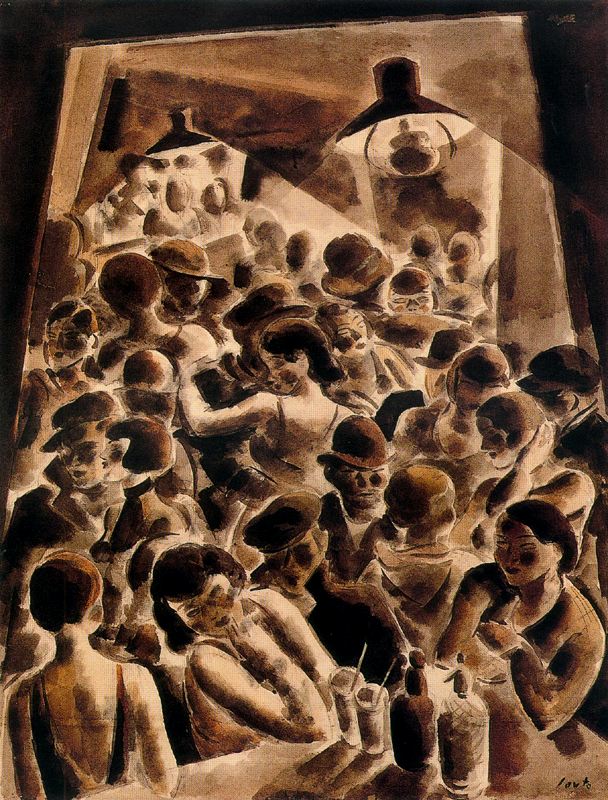This evocative piece of artwork, presumably a painting, captures the vibrant yet intimate atmosphere of a small, crowded nightclub or bar, reminiscent of a speakeasy. It appears to be heavily influenced by turn-of-the-century styles with elements from the 1920s, including the era's distinctive attire, with men sporting jackets and hats, and women in elegant dresses and low-backed gowns. The palette is predominantly various shades of brown—ranging from yellowish to reddish and maroon—alongside black and white, contributing to a monochromatic or sepia-toned effect. The scene depicts a bustling yet narrow room filled with animated interactions: men and women dancing closely, couples almost shoulder to shoulder, and groups gathered around tables or counters with elixirs and mixed drinks with straws. Notably, a woman at a table props up her head with her hand, drinks before her, while another woman across from her gazes intently. Another central figure, a woman with her eyes closed, dances with a partner, adding to the dynamic feel of the room. Overhead lighting illuminates parts of the scene, amplifying the room's lively ambiance. Intriguingly, a scrawled, unreadable artist's signature marks the lower right-hand corner. The entire composition, about five by seven inches in size, conveys a sense of bustling, working-class nightlife, filled with movement, chatter, and a palpable energy.